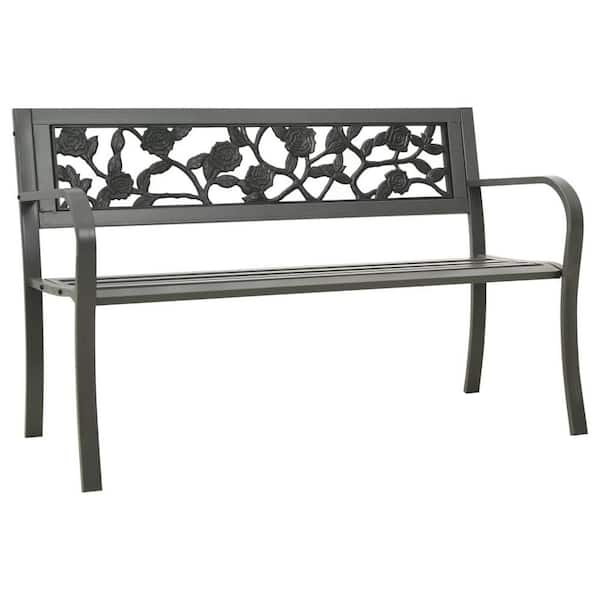This is an image of a contemporary outdoor bench, likely intended for backyard or garden use, though it could also be situated in a park. The entire bench is a solid gray color, possibly made from plastic or resin that is weather-resistant. The backrest features an ornate, cutout design of intertwined roses on vines, through which the background can be seen. This backrest design adds an elegant, decorative touch to the bench. The bench's seat includes horizontal slots, which add to its modern aesthetic. The arms of the bench are gracefully curved, extending down to the base, providing comfort and style. The bench is spacious enough to comfortably seat two to three people, and possibly up to four. This inviting piece would be perfect for relaxing outdoors, enjoying a cup of tea, or bird-watching. The image is presented against a plain white background, suggesting that it might be part of an advertisement.